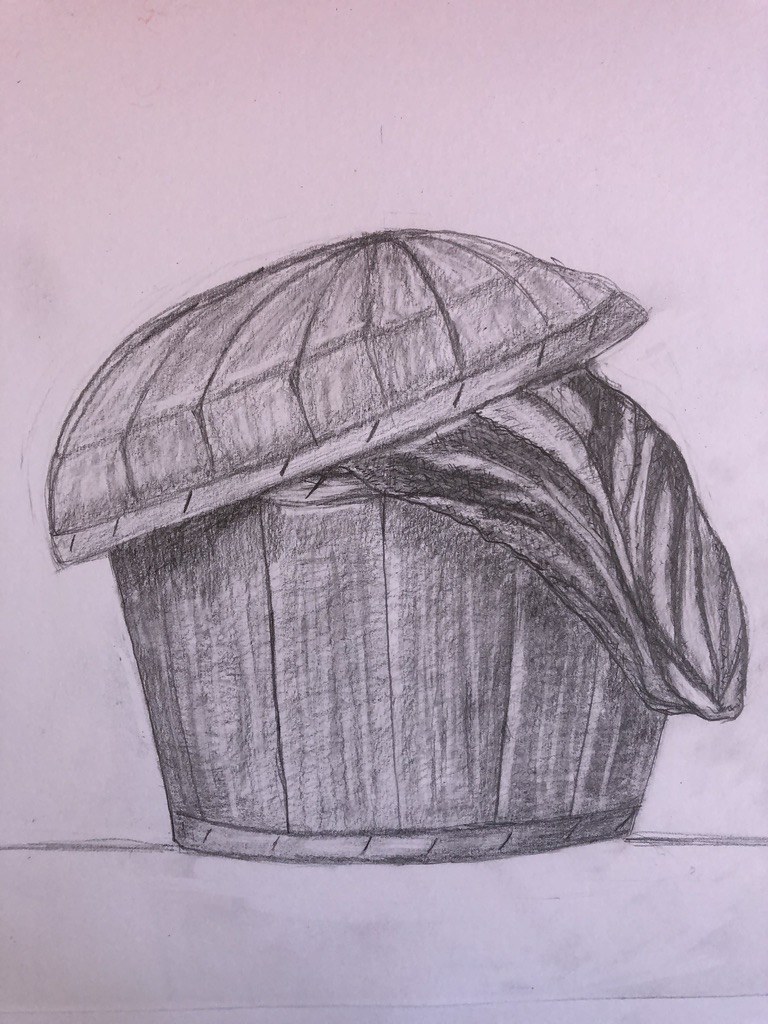This is a photograph of a detailed pencil or charcoal drawing on a piece of paper with a pink background that gradates to light purple towards the bottom. The focal point of the artwork is a barrel-shaped wooden basket with distinct texturing that reveals the wood's grain. The lid, a half-circle shape, is slightly askew and tilts to the left, detailed with individual wooden boards. Overflowing from the basket, a piece of fabric with zebra-like stripes hangs down to the right, appearing folded and scrunched up. The shading on the basket is dark and heavy, contrasting with the lighter pinkish tint of the paper. The image overall gives an impression of an art piece on a surface with smudged edges from the medium used. At the bottom, a line runs across, aligning with the barrel's base, adding to the composition's detail.